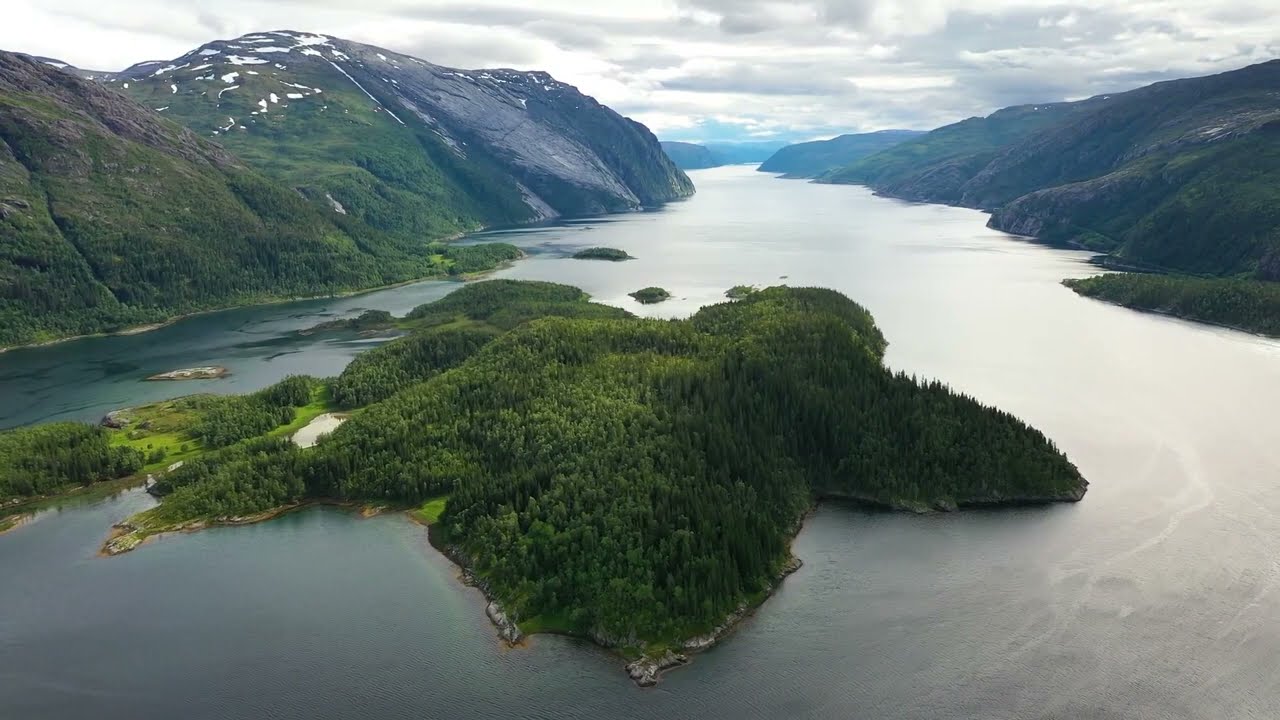The image depicts a breathtaking bird's eye view of a vibrant landscape featuring a wide river or inlet winding through a picturesque valley bordered by rolling, green hills. Dominating the center of the scene is a uniquely shaped, heavily wooded island, which appears uninhabited and resembles a starfish with its outstretched arms. This island is the focal point of the photo, surrounded by clear, flowing water that varies in hue from gray to blue. The river's channel is wider on the right side, facilitating open passage, while the left side appears narrower with potential shoals. The hills on either side boast lush greenery and rocks, while some peaks in the background exhibit patches of snow. Above, a blue sky adorned with a layer of white, fluffy clouds stretches across, and distant hills, tinged blue by atmospheric perspective, converge in the background.